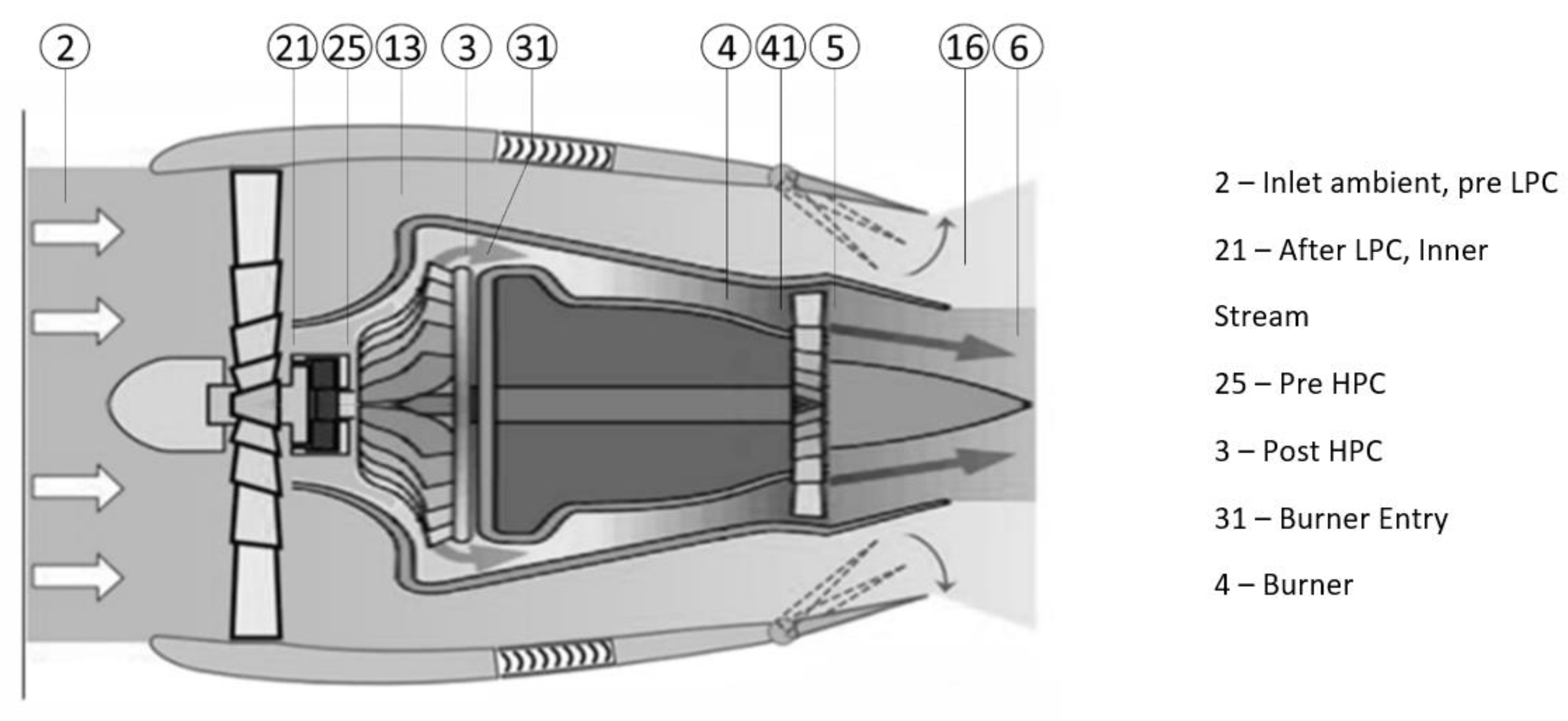This black and white illustration, in landscape orientation, is a detailed technical diagram of a jet engine. On the far left, a series of four white arrows point rightward on a gray background, labeled with the number "2" in a black text circle, indicating the inlet ambient pressure. Moving right, the engine's internal components are displayed in grayscale. The diagram showcases the fan with dark edge lines, followed by various grey-shaded mechanical sections, including the LPC (Low-Pressure Compressor) and HPC (High-Pressure Compressor). Numbered labels in white circles with black outlines, such as "21" for the inner stream after LPC and "31" for the burner entry, are connected to specific engine parts via lines. On the right-hand side, a column of text details these numbers: for instance, "2" corresponds to "Inlet Ambient Pre-LPC," "25" to "Pre-HPC," "3" to "Post-HPC," and "4" to "burner." The illustration, constructed in grayscale, captures the cutaway view of the jet engine with precise technical annotations and identifier bubbles aligned to each labeled component.